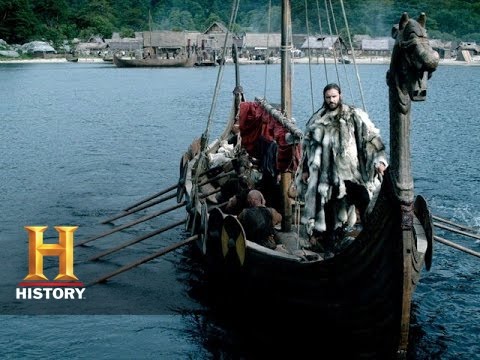The image is a photograph likely from a History Channel show, as indicated by the logo in the bottom left-hand corner: a large, golden, capital H with a red underline and the word "HISTORY" in white text beneath it. Dominating the scene is a Viking-style boat, its dragon-carved bow facing the camera. The vessel is long and narrow, with men rowing on either side using wooden oars—only the left rowers are visible. Each side of the boat features shields likely meant for protection against arrows. The boat also boasts a central mast stabilized by ropes, and an animal head carving—possibly a dragon or horse—at its top. Standing at the prow is a man in fur pelts, his long hair windblown. Behind the boat, approximately 200 meters away, lies a shore with a village and surrounding trees.